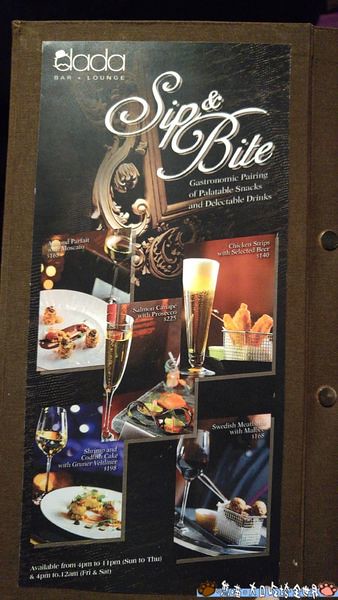The poster is mounted on a dark wooden wall, with a black background that enhances its visibility. The top half and part of the lower half of the poster feature a black background, lending a sense of elegance and sophistication. In the upper right corner, ornate white lettering spells out "Sip and Bite." Below this text, there is additional white lettering that is illegible due to its small size. 

In the top left corner, also against the black background, the words "Dada Bar and Lounge" are prominently displayed in white text. An ornate tan carved wooden picture frame peeks out from behind the "Sip and Bite" text, adding a touch of classical charm to the overall design.

The central portion of the poster is divided into five smaller images, each advertising different offerings available at the Bar and Lounge:

1. **Top Left Image**: This image is dark and features a white plate, though the specifics are hard to discern.
2. **Top Right Image**: A cup containing something fried is the focal point, accompanied by a beer to the left in a very tall pilsner glass.
3. **Center Image**: Overlapping the bottom right corner of the top left image and the bottom left corner of the top right image, this features two beer glasses on a reddish-brown background, with a plate of food situated between them.
4. **Bottom Left Image**: The top part of this image has a blue background. It showcases a wine glass on the left and a white plate with food.
5. **Bottom Right Image**: This image appears to feature sushi, complementing the other diverse food offerings.

More small writing appears at the bottom of the poster, but it is too small to read. This meticulously designed poster cleverly displays the variety of food and drink options available at the Dada Bar and Lounge, enticing potential guests with its elegant presentation.